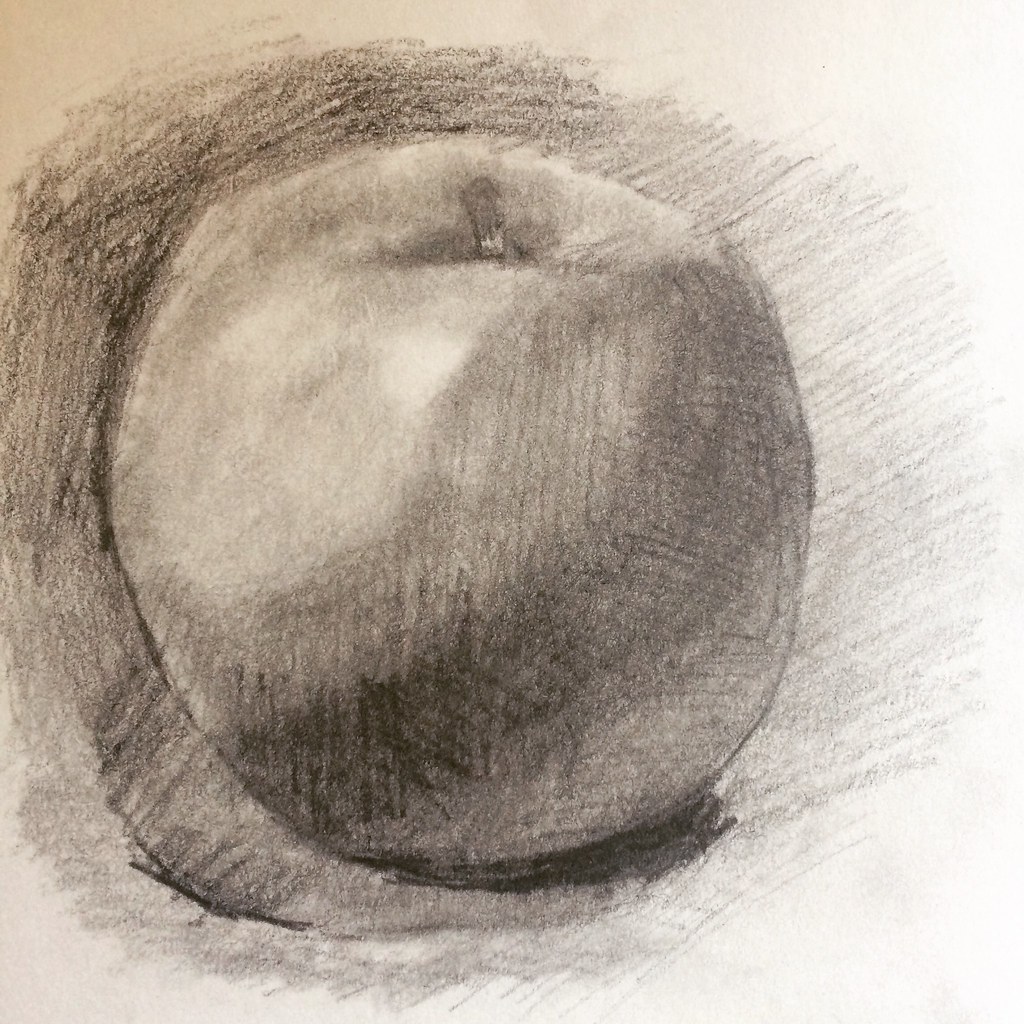The image captures a zoomed-in photograph of someone sketching an apple on a cream-colored piece of paper. The sketch, rendered entirely in pencil, features a circular, reasonably well-executed apple with a small stem protruding from the top. The artist appears to be diligently practicing shading techniques, as evidenced by the intricate play of light and shadow. Shading is prominently done along the left side of the apple, forming a c-shaped gradient that suggests a light source from the right. Additionally, there are subtle shadows around the stem and on the front left side, adding depth to the drawing. Although the sketch lacks the precision of professional artwork, it demonstrates considerable skill and learning progress. The black-and-white sketch showcases a shiny highlight on the apple, typical of how light reflects off its surface, further emphasizing the artist's efforts to capture realistic details.